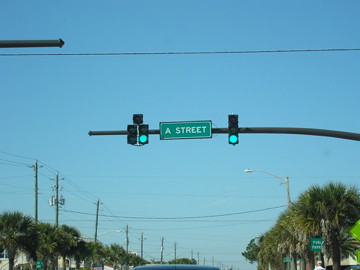This photograph, taken from the passenger seat of a vehicle, showcases a street intersection on a clear, sunny day. Dominating the frame is a long, dark gray metal pole supporting two traffic lights and a green street sign with white lettering that reads "A Street." The traffic lights, unusually black in color rather than the typical yellow, are illuminated green, signaling that traffic may proceed. Lining both sides of the street are rows of vibrant, green-leaved trees, their branches spreading out beneath a pristine, blue sky. Overhead, numerous power lines crisscross the road, adding a complex web of lines to the otherwise serene and orderly streetscape.